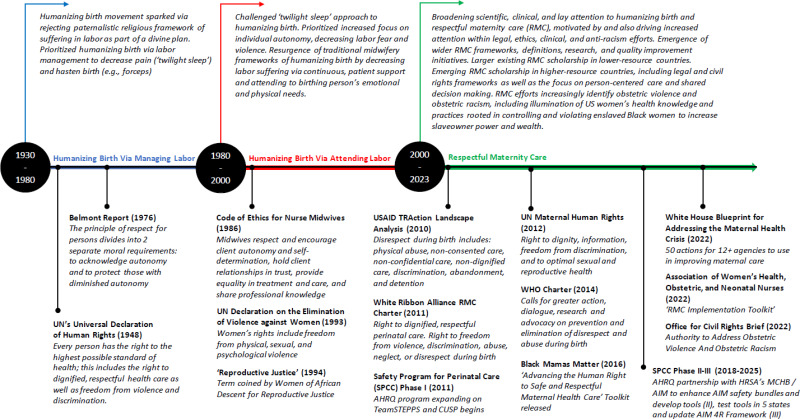The image presents a detailed grid illustrating the evolution of childbirth from 1930 to 2023 against a white background with no border. A prominent horizontal black line divides the image into two sections, representing a timeline of significant periods in childbirth history. At the top, three black circles denote different eras: "1930 to 1980" on the left, "1980 to 2000" in the center, and "2000 to 2023" on the right. Each circle has a corresponding blue, red, or green arrow above it pointing right, indicating progress over time.

Beneath the black line, each era is expanded upon with detailed text. 

- The left section, marked by the years 1930 to 1980, highlights the "humanizing birth movement" sparked by a rejection of the paternalistic religious framework that saw suffering in labor as part of a divine plan. Key developments listed here include the 1976 Belmont Report and the UN's Universal Declaration of Human Rights.

- In the center section, covering 1980 to 2000, significant points include the establishment of a code of ethics for nurse midwives and the emergence of reproductive justice initiatives.

- The right section, spanning 2000 to 2023, details advancements in maternal human rights, the implementation of the WHO Charter, the Black Mamas Matter initiative, and the safety program for perinatal care.

The text in the image is written in both blues and blacks, and despite its small size, it is organized into paragraphs and bullet points for clarity, depicting how childbirth practices and ethics have evolved over nearly a century.